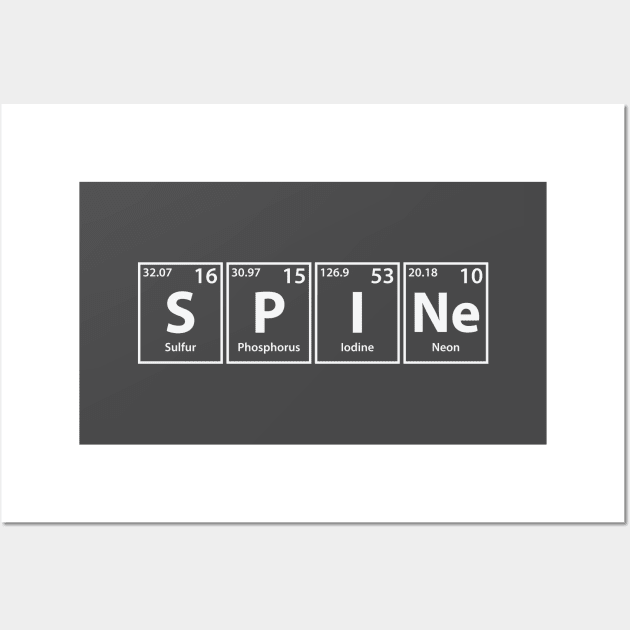The image features a gray background bordered by a thick white rectangle, which in turn is surrounded by a dark gray rectangular frame. At the center of this layout are four individual squares arranged to spell out the word "SPINE" using elements from the periodic table. Each square resembles a Scrabble tile but contains detailed information akin to periodic table notation.

The first square shows a white "S" standing for Sulfur, with the atomic number 16 and an atomic weight of 32.07. Following it, the second square displays a white "P" for Phosphorus, marked with the atomic number 15 and an atomic weight of 30.97. The third square features a white "I" representing Iodine, labeled with the atomic number 53 and an atomic weight of 126.90. Lastly, the fourth square combines "N" and "e" for Neon, indicating the atomic number 10 and an atomic weight of 20.18. Each element is presented in a manner similar to its appearance on the periodic table, encapsulated in individual boxes.